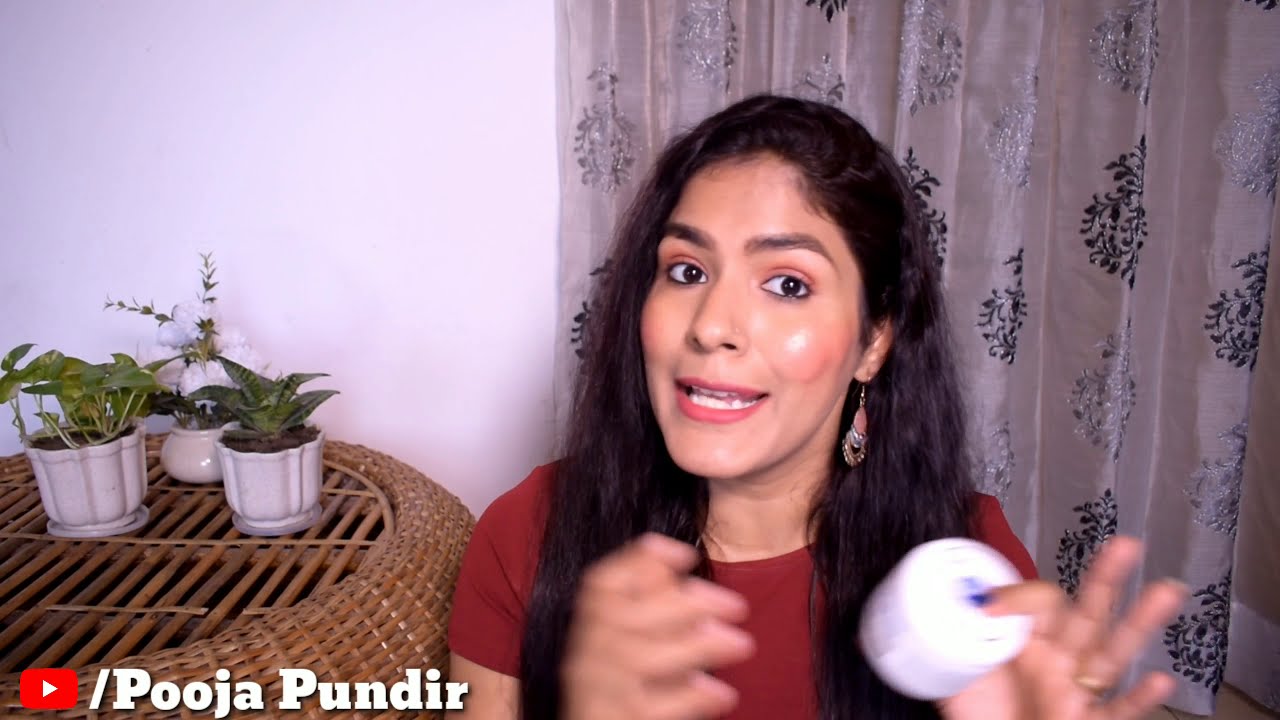This is a landscape-oriented freeze-frame from a YouTube video featuring a young South Asian woman, likely Indian or Pakistani, named Pooja Pundir. She is positioned centrally in the image, facing the camera and speaking with her hands in motion, suggesting she is gesturing as she talks. Pooja has long, dark brown hair flowing over her shoulders, light skin, and is wearing a red short-sleeve shirt. One visible earring dangles in a teardrop shape from her ear. In her left hand, she holds a roll of white receipt paper, and a wedding band is visible on that hand.

Behind her, the wall is white, and a sheer grayish curtain with a black repeating floral or fern design adds texture to the background. To her left, there is a wicker table adorned with three small white pots: one contains a vine plant, another appears to be a succulent, and the third's identity is unclear. At the bottom left corner of the image, the YouTube logo is accompanied by the text "Pooja Pundir" in a bold, upper and lowercase sans-serif font, presumably her YouTube handle.